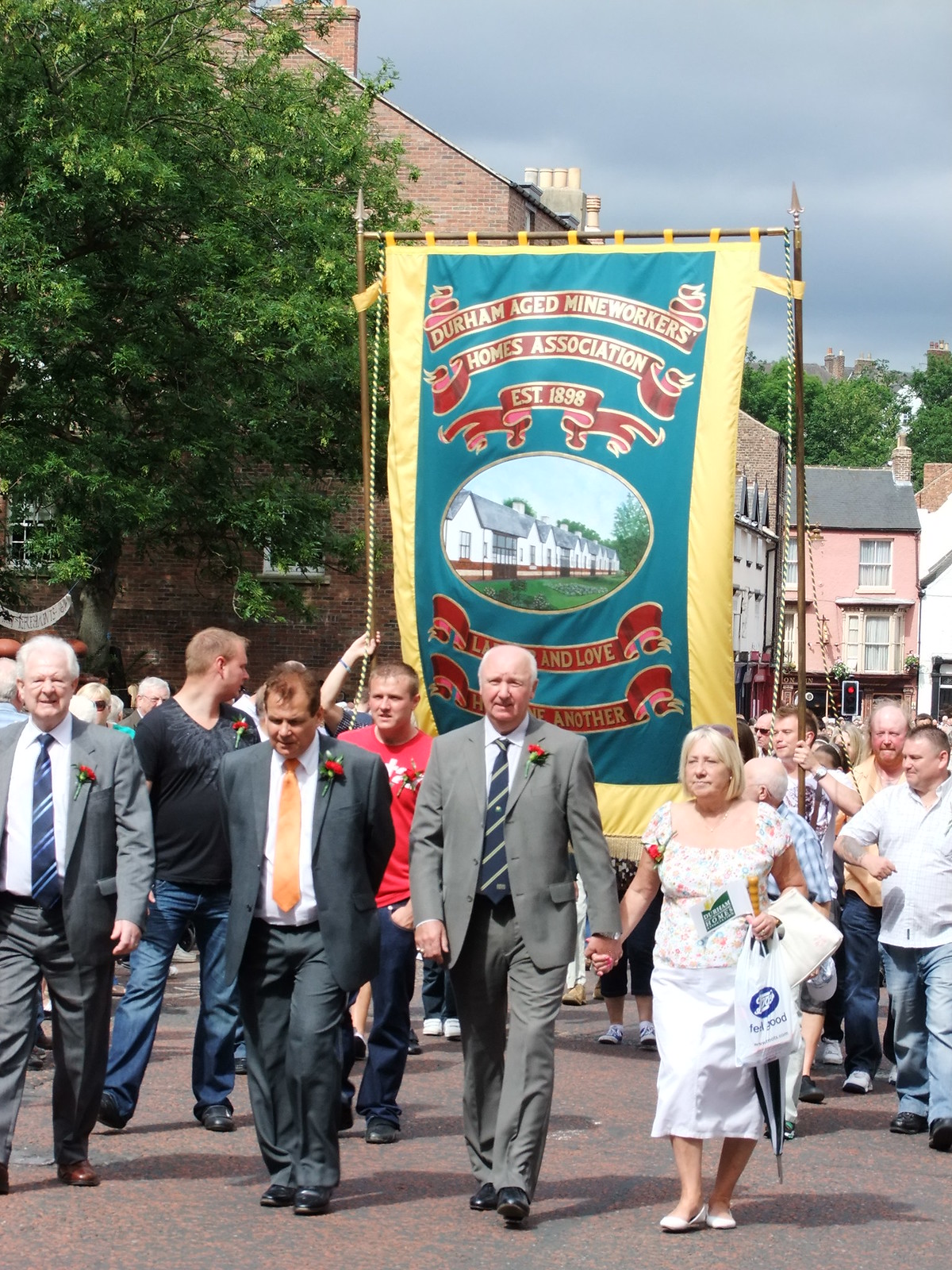This is a photo of an English parade with a mix of older and younger people marching towards the camera. In the front, several individuals in business suits are visible. From left to right, there is an older man in a business suit, followed by a somewhat younger man, also in a suit, and another older man holding hands with a woman presumed to be his wife. The older man has a gray suit, a black tie, a white shirt, and a red rose in his breast pocket. The woman, dressed in a white dress with little red dots, carries a grocery bag, a purse, and an umbrella. Beside them is another man in a black suit with an orange tie, looking down.

Behind them, a large and vibrant banner is displayed, nearly the size of three people in length and much taller. The banner reads "Durham Aged Mine Workers Homes Association established 1898," surrounded by colorful decorations in gold, red, blues, and greens, with a detailed depiction of houses in the center. Although partially obscured by the crowd, additional text on the banner mentions themes of love. The scene is outdoors on an overcast day, with shadows stretching long behind the marchers, suggesting it's later in the day. The parade likely celebrates a retirement home for mine workers, highlighting the community's support and appreciation for their contributions.